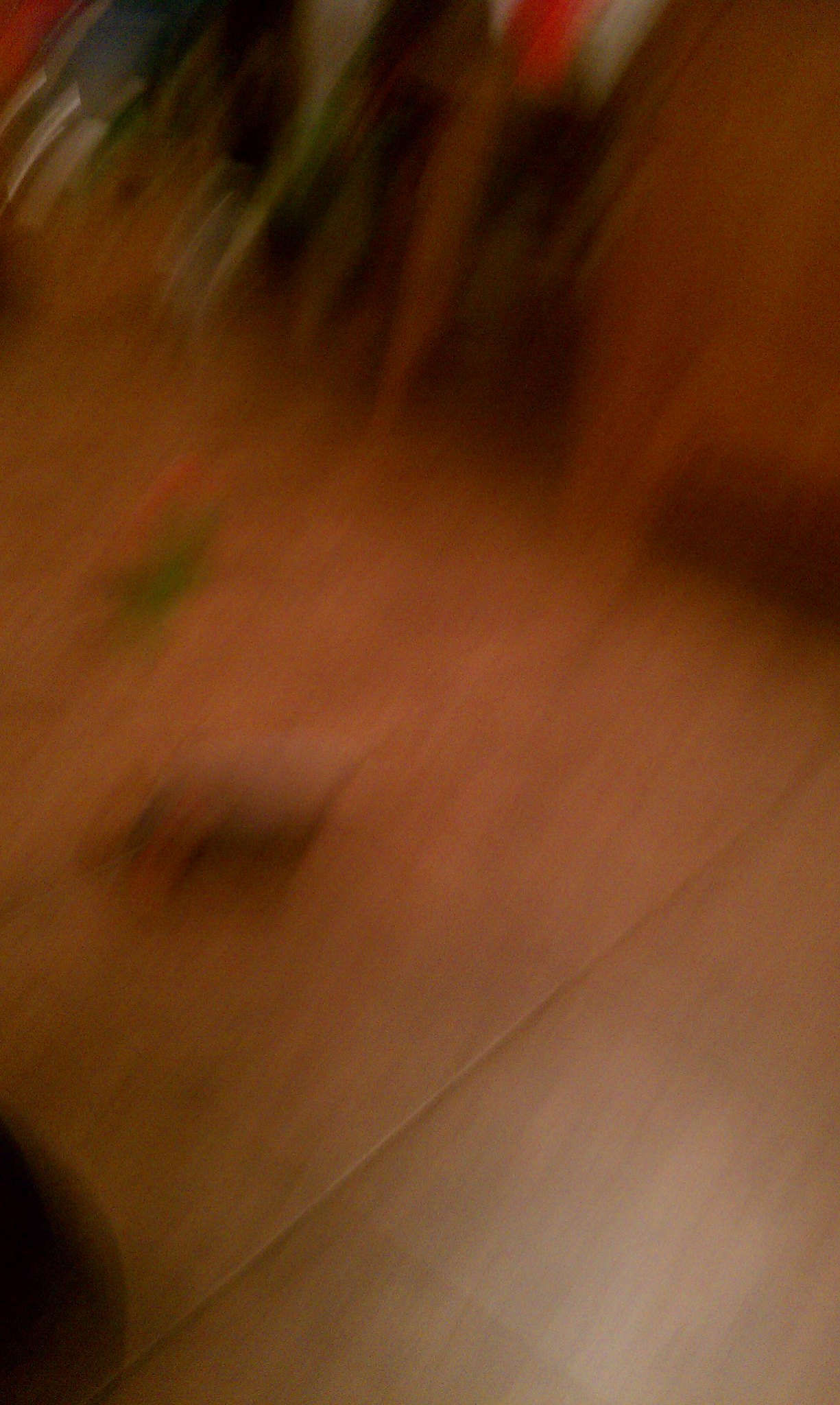The image depicts a blurry indoor scene that is difficult to make out due to significant distortion. The floor is covered with large tiles and a small, indiscernible grayish animal, likely a small dog, is present near the center. Adjacent to this animal is something green, possibly a plant with a hint of pink at the top. To the right, a wall is faintly visible, and in the background, there seems to be some furniture, perhaps a table, positioned at an angle that complicates visibility. The left side of the image shows metal pipes. The scene might be captured at night given the dark background.